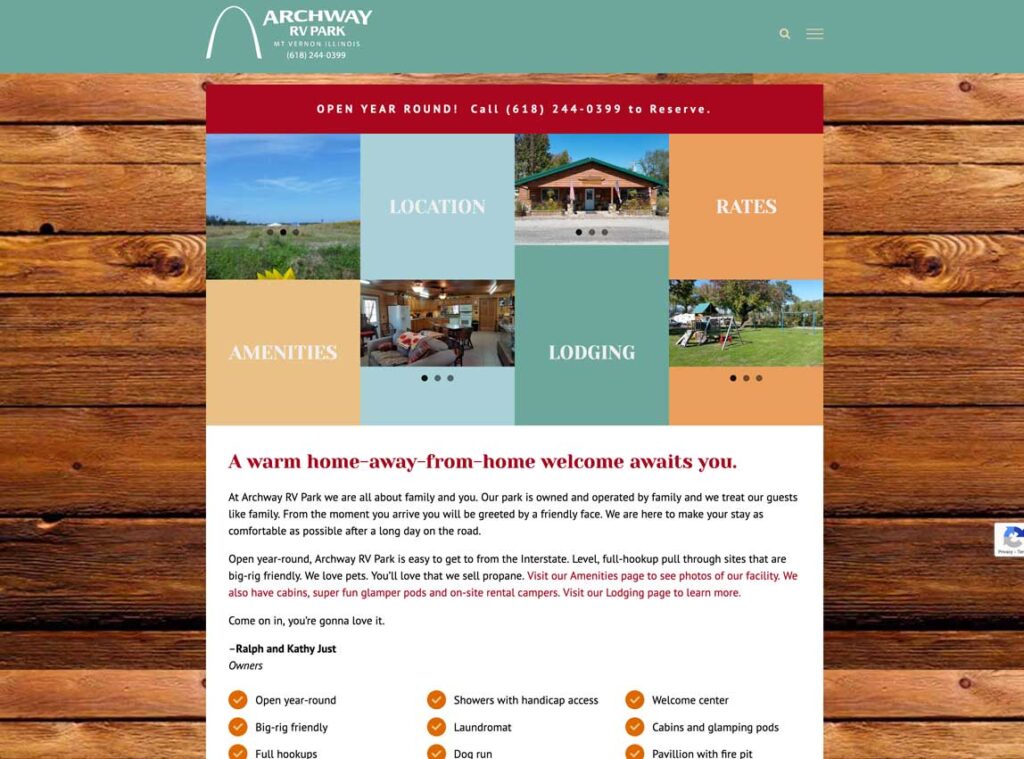Detailed Caption:
The image features a light blue banner at the top, prominently displaying the name "Archway RV Park" in a bold white font. Beneath this, a striking white arch serves as a visual marker. To the right of the arch symbol are three common website icons: a magnifying glass for search, and three horizontal lines indicating a menu.

Highlighted in red, the text "Open Year Round" draws immediate attention, followed by an invitation to call "615-244-0599 to reserve." Below this information, the image transitions into a lush, green grassy area bathed in daylight, giving a welcoming view of the RV park's front entrance.

To the right of the grassy image, large text reading "Location" helps visitors identify the feature of the scenery. Moving further to the right, an orange section labeled "Rates" sits adjacent to a lighter orange box titled "Amenities," which displays a photograph showcasing some of the park's available facilities.

Continuing down, a light green box signals the "Lodging" section. Next to it, an orange box includes another scenic outdoor image adorned with greenery, accompanied by the warm message: "A warm home away from home welcome awaits you." This area emphasizes family-oriented hospitality, stating that Archway RV Park is family-owned and operated, committing to treat guests like family from the moment they arrive.

The caption reiterates that Archway RV Park is open year-round, easily accessible from the interstate, and boasts well-maintained, level, full-hookup pull-through sites accommodating large rigs. Pet-friendly policies are highlighted, along with available amenities such as propane sales. The caption encourages visitors to explore the Amenities page for more facility images and mentions additional lodging options like cabins, glamper pods, and onsite rental campers, directing them to view the lodging page for further details.